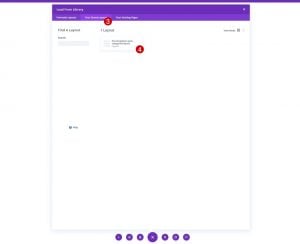The image features a small and somewhat illegible user interface, primarily characterized by purple accents against a white background. Across the top, from the upper left to the upper right, is a long, thin purple line. Below this, a pop-up menu dominates the scene, with its header stripe colored in purple, though the text within this header is unreadable due to the image's diminutive size.

Directly below the header, there appears to be a lighter purple stripe featuring three tabs, with the middle tab highlighted. Near this highlighted tab, there is a red circle enclosing the number three. The rest of the menu is populated with text that remains unreadable, consisting of two sections with words on the left and right sides. Additionally, there is a red circle containing the number four, drawing attention to the menu's lower section. 

At the very bottom of this pop-up menu, there are several small purple circles arranged in a horizontal row. These circles are numbered sequentially, from one to seven. Notably, the fourth circle is larger than the others, indicating that it could currently be selected, suggesting a pagination system where the viewer is on the fourth page.

Overall, the image seems to highlight specific elements of the user interface, marked by numbered red circles, but the text and finer details remain too small to decipher.